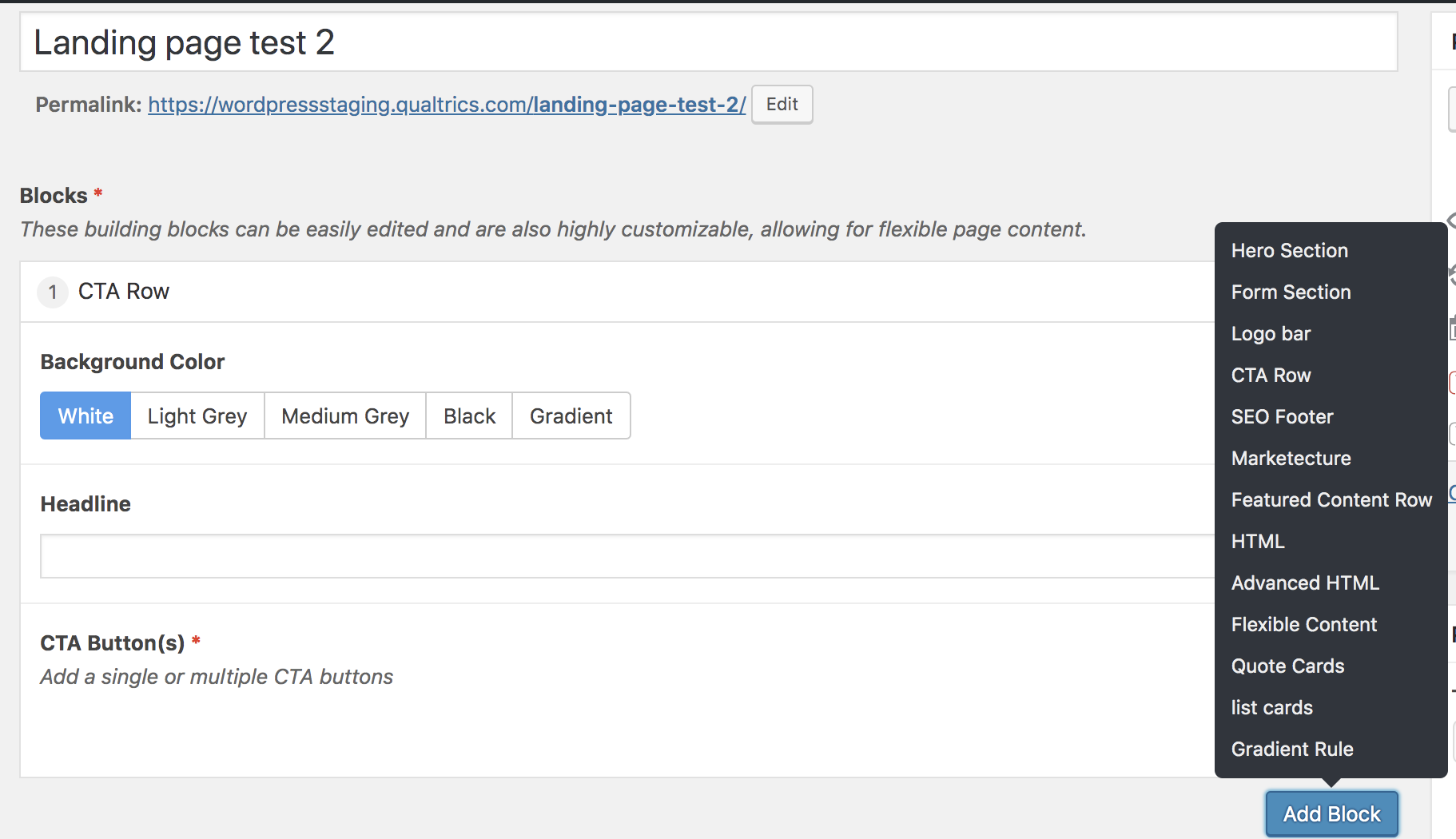This image depicts a section of a webpage with a light gray background. At the top, there's a long white box labeled "Landing Page Test 2." Below this, a web address including the term "wordpressing" is displayed, though it's worth noting that the word "pressing" is misspelled with an extra 's'. This address is clickable and editable.

The page features a section titled "Blocks" marked with orange asterisks. An accompanying description reads, "These building blocks can be easily edited and are also highly customizable, allowing for flexible page content."

A prominent Call-To-Action (CTA) row is centered on the page, identified by a light gray circle with the number '1' inside it. The background color options for this section include light gray, medium gray, black, and gradient, with blue and white highlighting.

Additionally, there's a headline box consisting of a long, empty white rectangle. Further down, more CTA buttons are offered, again marked with orange asterisks and the text, "Add a single or multiple CTA buttons."

On the right-hand side, a pop-up is visible indicating that someone clicked "Add Block." This pop-up is blue and displays a black box with numerous selectable options for adding new blocks to the webpage.